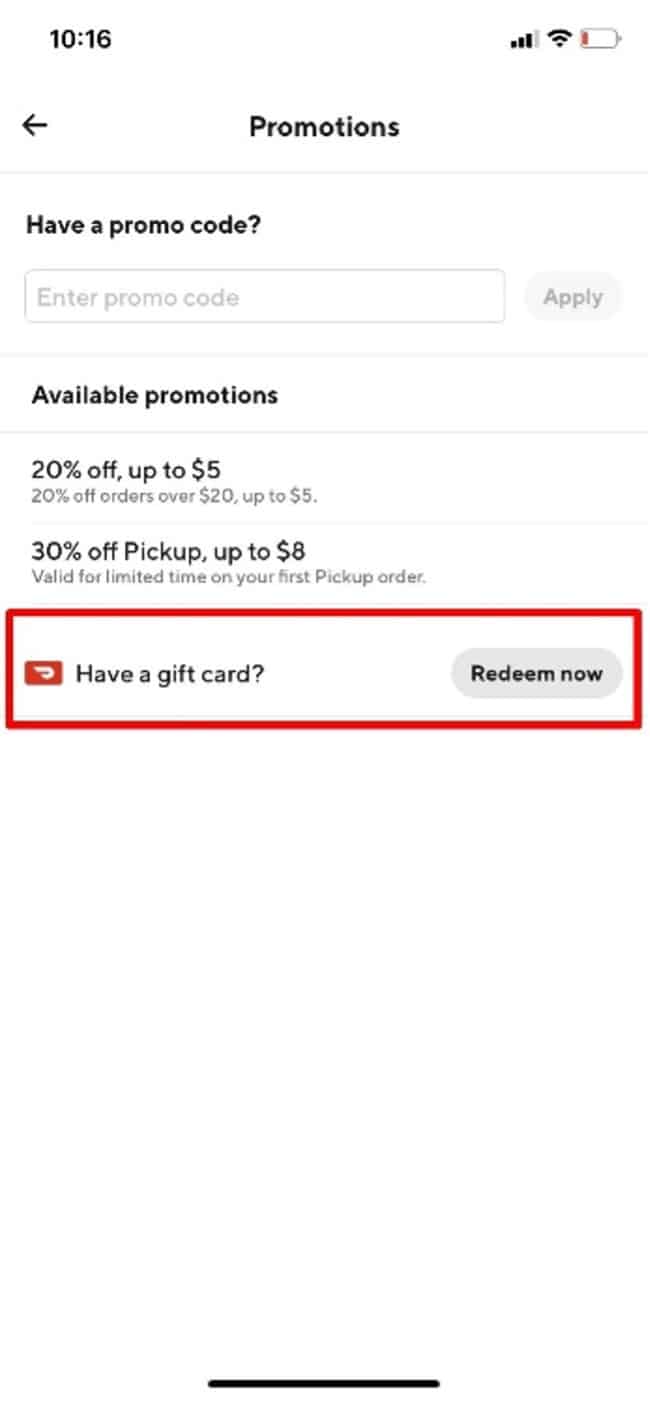Screenshot of a mobile screen displaying DoorDash promotions at 10:16 AM. The interface shows three bars of mobile service, full WiFi connectivity, and a nearly depleted battery indicated by a red bar. 

Below, there's a navigation arrow pointing left and the text "Promotions" centered at the top. A grey horizontal line segments the screen below this. To the left, it prompts with "Have a promo code?" followed by a grey outlined box for entry labeled "Enter promo code" and a greyed-out "Apply" button on the right.

Another grey line divides the section below which shows "Available Promotions" in bold, followed by additional promotions separated by grey lines. These promotions include: 
- "20% off up to $5"
- "20% off orders over $20 up to $5"
- "30% off pickup up to $8, valid for limited time on your first pickup order"

At the bottom, there is a box outlined in red with a DoorDash icon, captioned "Have a gift card?" Inside this box is a greyed-out oval button labeled "Redeem Now." The lower portion of the screen features blank white space ending with a short black line at the bottom. The screenshot appears to be from DoorDash, with both DoorDash promotions and gift card inquiry elements visible.